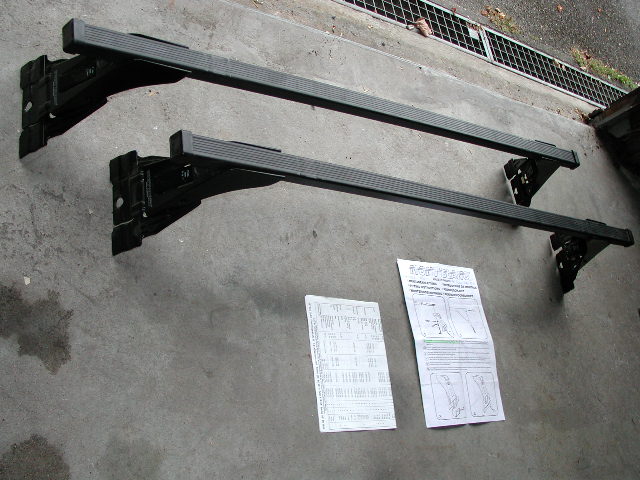The photograph depicts two black roof rack crossbars positioned on a concrete surface, likely at the entrance of a garage. The crossbars, which show a textured or wavy rubber lining on their tops, are nearly parallel but slightly offset from each other. In front of the crossbars lie two pieces of paper: a larger one, presumably an instruction sheet for installation, and a smaller one, potentially a receipt or warranty information. Beyond the concrete floor, a metal drainage grating is visible, with a sliver of grass peeking through, suggesting the outdoor boundary of the garage.